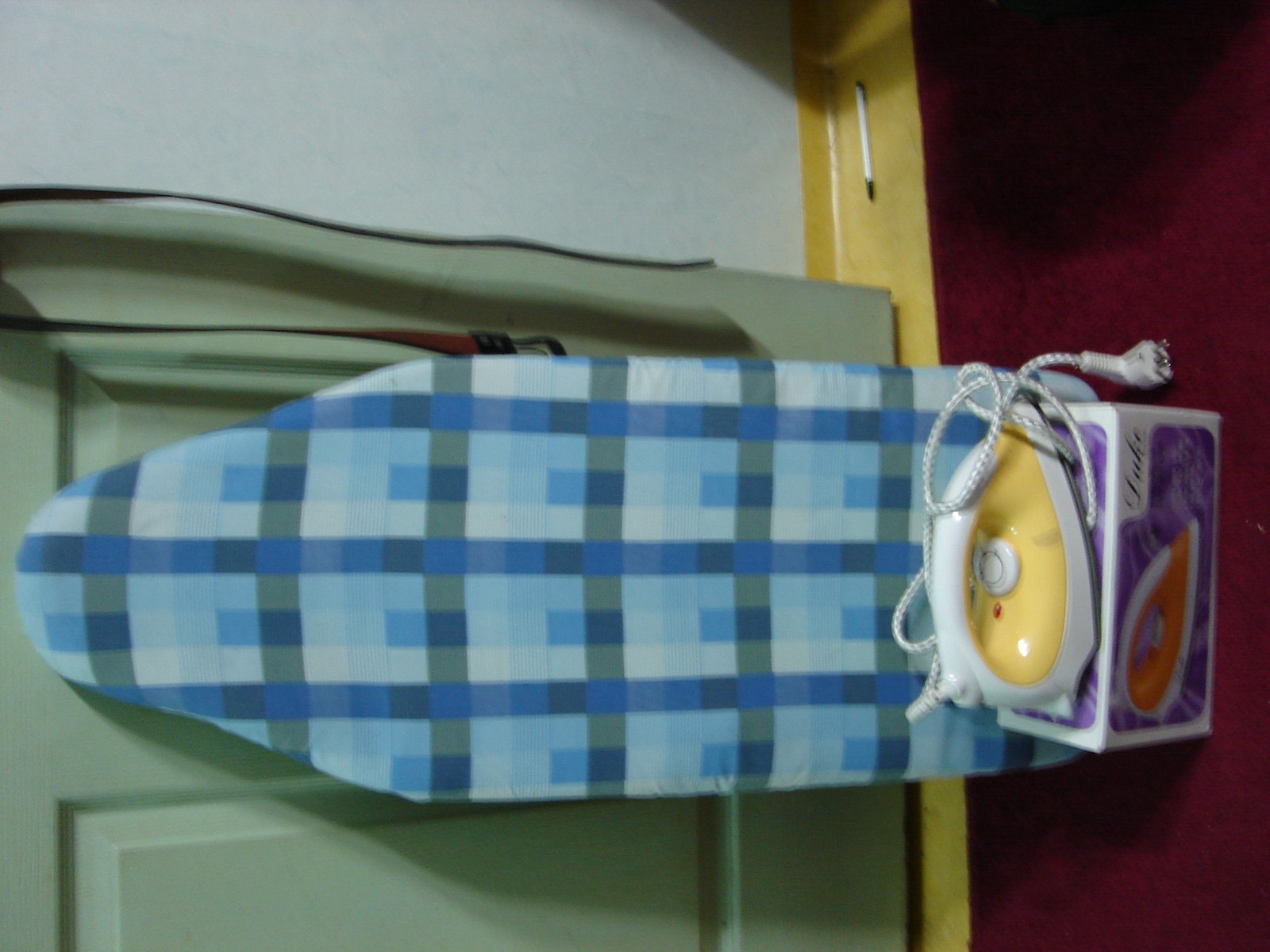This sideways photograph, taken indoors, showcases a room with a maroon carpet and off-white walls that have a yellow border near the floor. A light green door is visible, with a brown belt hanging from its doorknob. Leaning against the door is a plaid-patterned ironing board featuring a mix of white, gray, light blue, and dark blue squares. In front of the board, there is a white and purple box with a picture of a red iron on it. Atop the box sits an actual iron that closely resembles the one in the picture, except it has a yellow body. The iron comes with a white handle, white base, white dial, and a white power cord.